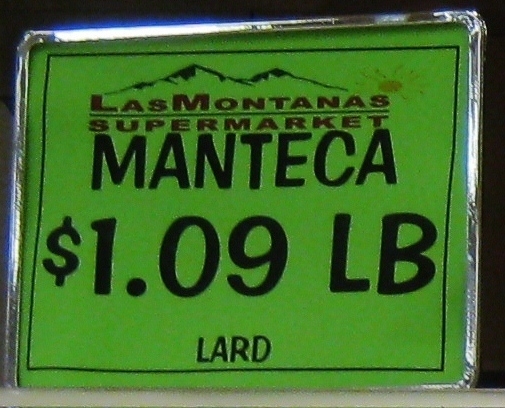The image captures a promotional sign displayed in a grocery store. The sign, which has a distinctive metal outline resembling a license plate, is primarily bright green with a thin black border around the edges. Inside the sign, at the top, is a logo featuring mountains with a sun in the background, and text that reads "Las Montanas Supermarket" (notably missing a tilde in "Montanas"). Below the supermarket name, there is a large, prominent price of $1.09 per pound for "Manteca" (lard), with the word "LARD" spelled out at the very bottom in small letters. The sign is propped up against a black backdrop, making the colors and details stand out vividly.